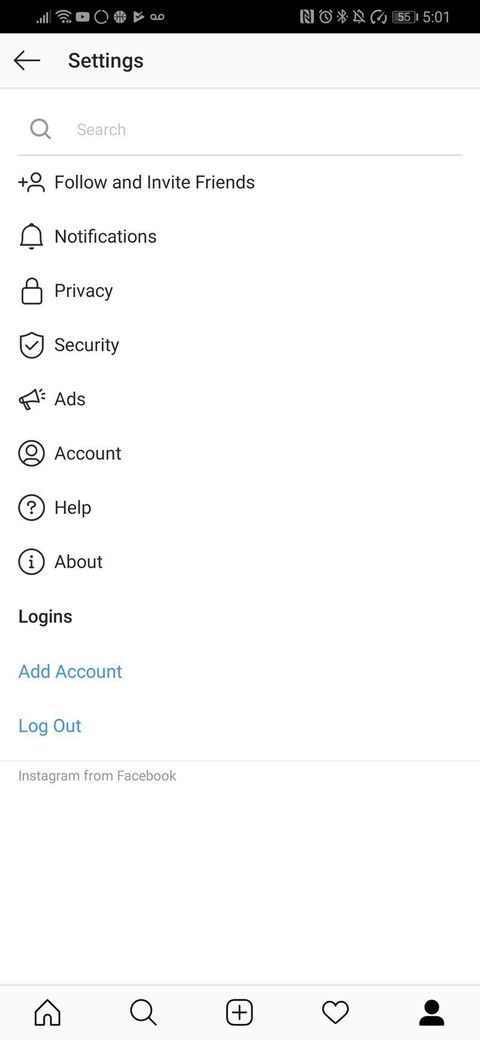The image depicts a smartphone screen showing a settings page. At the top, a thin black ribbon displays several icons on the left, including symbols for voicemail and YouTube. On the right of this ribbon, the time is shown as 5:01, along with icons indicating the phone is silenced and some other unidentified icons.

Below this, a light gray ribbon features the word "Settings" in black text, accompanied by a black back arrow on the left. The main content of the screen is set against a white background. At the top, there is a light gray search magnifying glass icon, followed by the word "Search" in gray text, and a faint gray line runs horizontally across the page.

Following these elements, a vertical list of options in black text is presented. The options include "Follow and Invite Friends," "Notifications," "Privacy," "Security," "Ads," "Account," "Help," and "About." Additionally, the word "Logins" is displayed in bold black text. Beneath this, "Add Account" in bright blue and "Logout" are listed.

At the bottom of the screen, another light gray ribbon contains icons representing different functions from left to right: Home, Search, Add, Favorite, and People or Contacts.